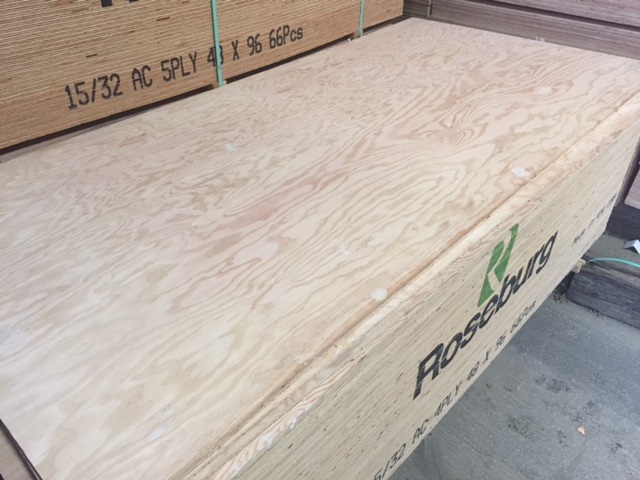The image depicts a warehouse setting with a concrete floor. In the foreground, there is a large, light blonde plywood box bearing the name "Roseburg" and a logo consisting of a big green "R" on its side. This box appears to have indentations indicating its wooden texture. Behind it, another large, darker wood box is visible, adorned with green zip ties that likely seal it. This darker box has various detailed markings, including "1532 AC 5 ply," and partially obscured numbers and letters such as "48" or "40," alongside "X 9666 PCS." These inscriptions potentially denote dimensions and shipment tracking information. The overall scene suggests an organized storage area involving substantial wooden crates used for logistics or storage purposes.